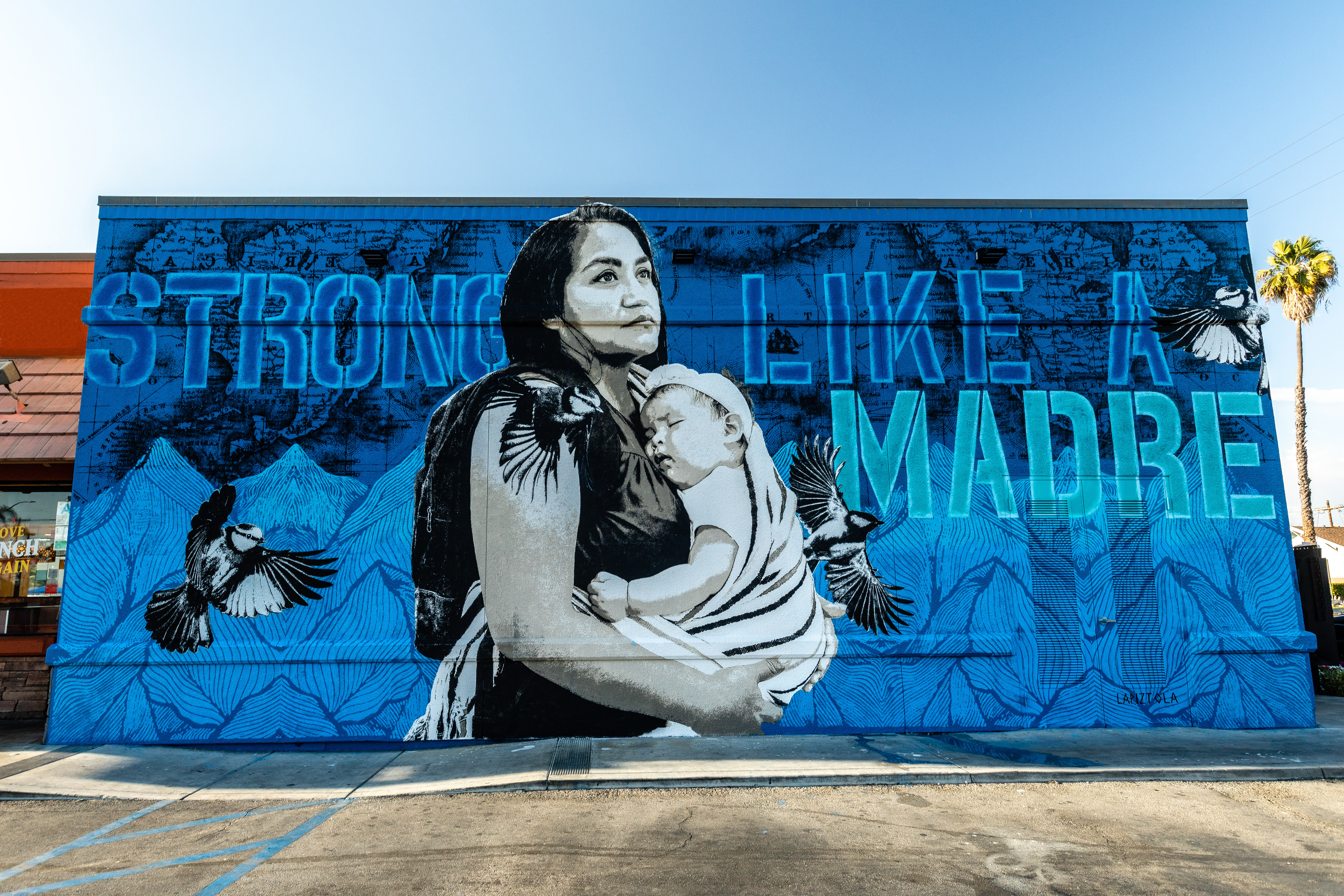The mural, painted on the side of a building, is a detailed, captivating piece featuring various shades of blue as its primary color. The bottom half of the mural is a light blue depicting a mountainous landscape, while the top half transitions into a darker blue featuring map-like elements. Central to the mural is a powerful, monochromatic depiction of a woman with black hair and eyebrows, holding a sleeping baby nestled against her chest in a ring sling. The mother's expression is pensive, and she gazes upward, embodying strength and resilience. Above them, in large, bold blue letters with white shadowing, the words "Strong like a Madre" convey a message of maternal strength. The mural also includes three birds: one flying in the mountainous area on the left, another near the map at the top, and a third appearing to soar in front of the mother. Adding to the tropical ambiance, a palm tree is visible on the right-hand side of the mural, with an adjacent parking lot and an orange building nearby, indicating a vivid setting.